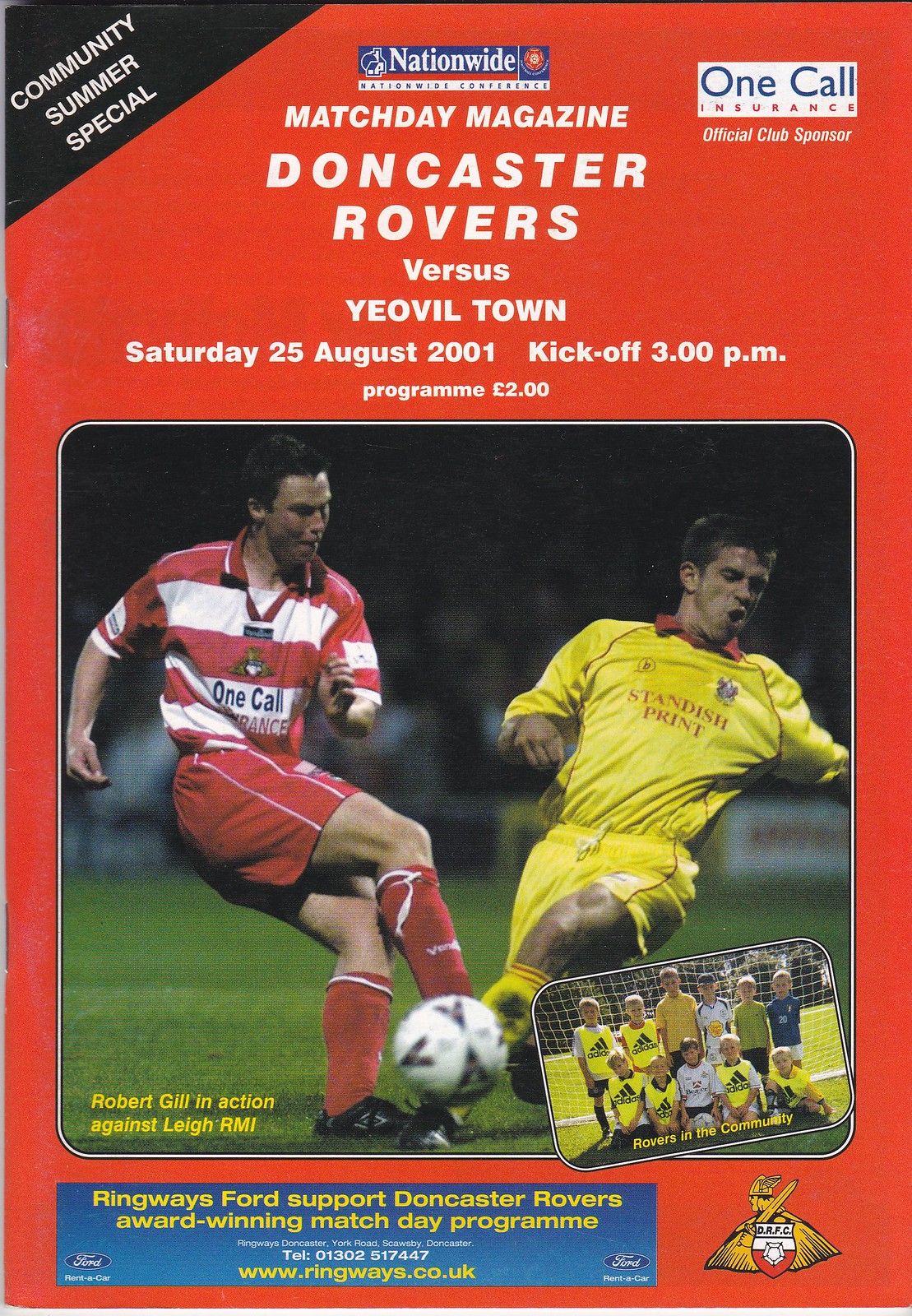The image is a highly detailed cover of a Match Day Magazine for a soccer game between Doncaster Rovers and Yeovil Town, scheduled for Saturday, 25 August 2001, at 3 p.m., with a program cost of 2 pounds. The entire background is a striking red. In the top left corner, a black triangle with white text reads, "Community Summer Special." The top section is filled with white text: "Match Day Magazine, Doncaster Rovers versus Yeovil Town, Saturday, 25 August 2001, kickoff, 3 p.m. Program, 2 pounds." On the upper right, there's a white rectangle with blue text reading "One Call Insurance," labeled as the official club sponsor.

Dominating the center of the cover is a dynamic action photograph of two soccer players: one on the left, clad in a red and white horizontally striped shirt, red shorts, and red socks, tussling for the ball with a player on the right dressed head-to-toe in yellow. The caption in yellow text reads, "Robert Gill in action against Leigh RMI." There is also an inset photograph of a group of children posing in front of a soccer net, captioned "Rovers in the community" in yellow text. 

The bottom left features a blue box with yellow text promoting "Ringways Ford," supporting Doncaster Rovers' award-winning Match Day Program, followed by a contact number and website. The bottom right displays the Doncaster Rovers logo: a man with a sword on his shoulder, set against a shield bearing the letters "DRFC" and a small rose design.